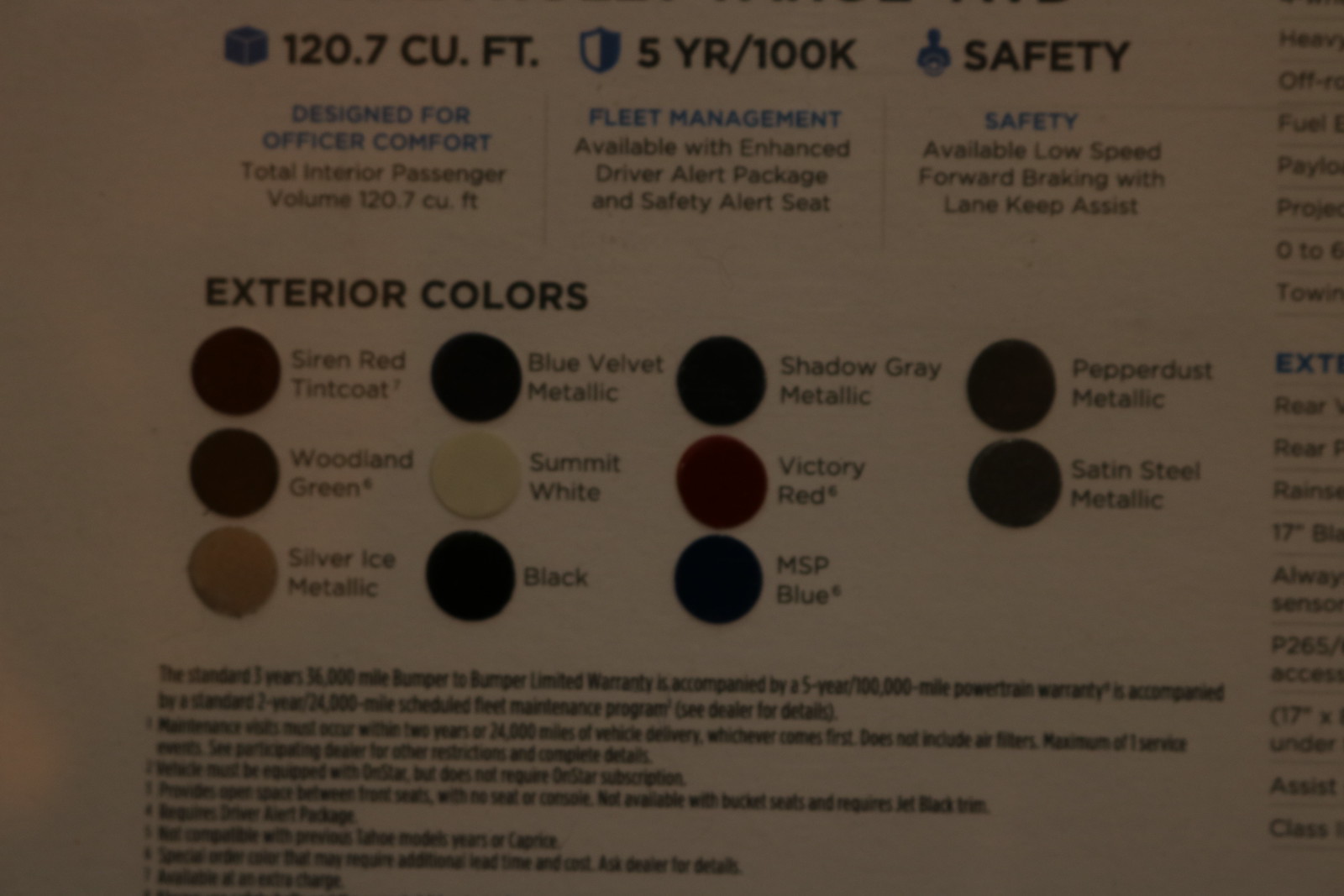The image appears to be a section from a car brochure, possibly a page from a magazine. The top section prominently displays the interior space of the vehicle, highlighting "120.7 cubic feet." Adjacent to this, a shield icon indicates a "5 years / 100K" warranty. Next to this, an illustration of a person emphasizes safety, stating "safety available lower speed for braking with lane keep assist." Below these headings, there are detailed paragraphs outlining various features: "Designed for officer comfort with a total interior passenger volume of 120.7 cubic feet," "Fleet management available with enhanced driver alert packages and safety alert seat," and the aforementioned safety features.

Further down, there's a section titled "Exterior Colors," listing various color options such as "Siren Red Tintcoat, Woodland Green, Silver Isotalic, and Blue Velvet Metallic," each accompanied by a circular swatch. This segment is visually organized in columns, with three rows of color samples—each color represented by a dot and labelled accordingly.

The bottom portion of the image contains small text, likely footnotes, providing additional details likely related to the vehicle’s features and offers. The overall image is poorly lit, contributing to a somewhat unclear view of the details, suggesting it may have been taken in suboptimal lighting conditions.